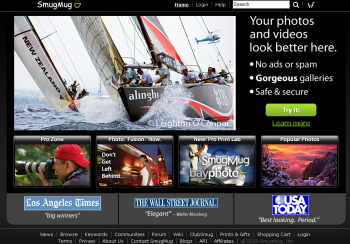In this screenshot set against a predominantly black background, the website name "SmugMug" is visible in the top left corner. The upper right side features a search bar iconified with a magnifying glass, followed by a shopping cart icon. Below this search bar, there is gray text stating: "Your photos and videos look better here." There are three accompanying bullet points: "No ads or spam," "Gorgeous galleries," and "Safe and secure." A prominent green action button with "Try it" inscribed is situated immediately below the text.

Central to the visual appeal, a striking, full-color photograph depicts sailboats gracefully navigating a body of water, either a river or the ocean. One of the sailboats prominently displays the word "Alingu" on its front in white text. Above the sailboats, in the upper right corner of the image, a helicopter hovers in mid-air, seemingly observing the maritime activity below. The overall composition is designed to be both visually engaging and informative, emphasizing the platform's features and calling viewers to action with its clear and attractive layout.